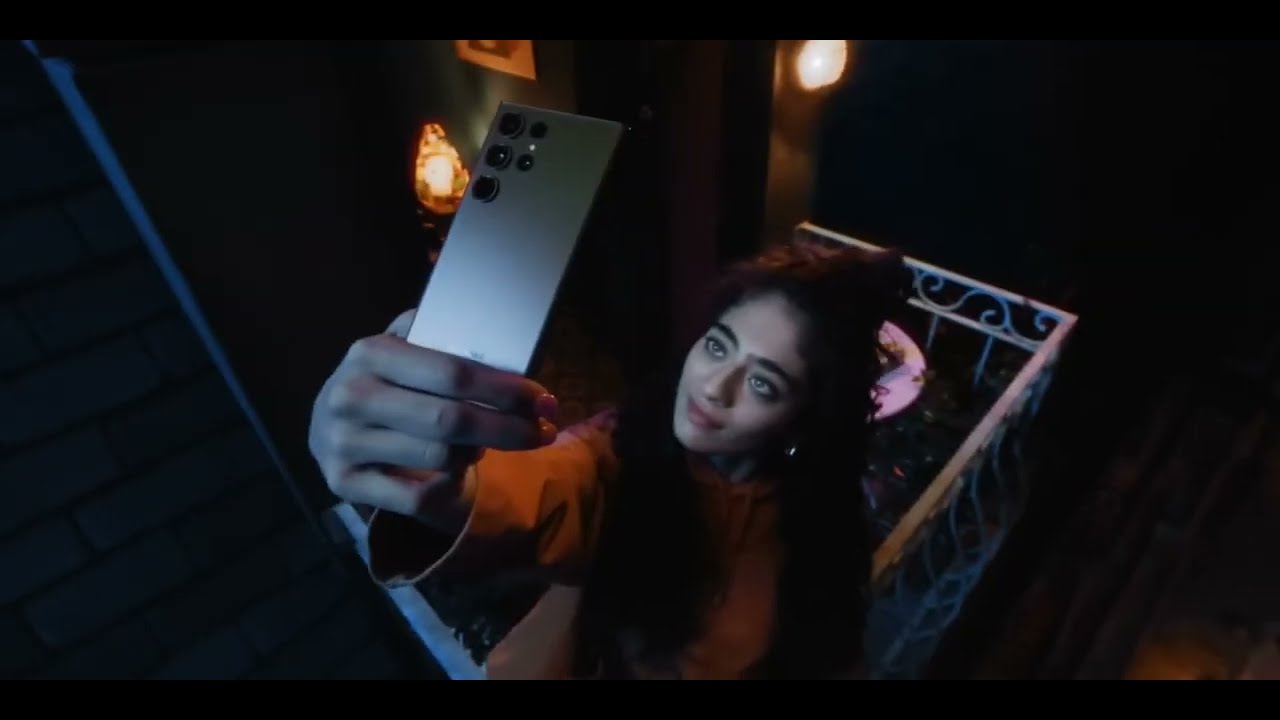This photograph captures a woman standing on a balcony at night, taking a selfie. She is holding her phone high above her head with her thumb and two fingers. The balcony features a wrought iron gate with a swirly design and a white, round table with something on it. The woman has long, wavy dark hair, some of which is piled on top of her head, and she is smiling. She is wearing a red shirt and pink lipstick, with a hint of shine visible from an earring. Behind her, the background reveals a well-lit room through a window, showcasing green walls, a painting, and other illuminated furnishings. Additionally, there is a lamp affixed to the exterior wall near her.